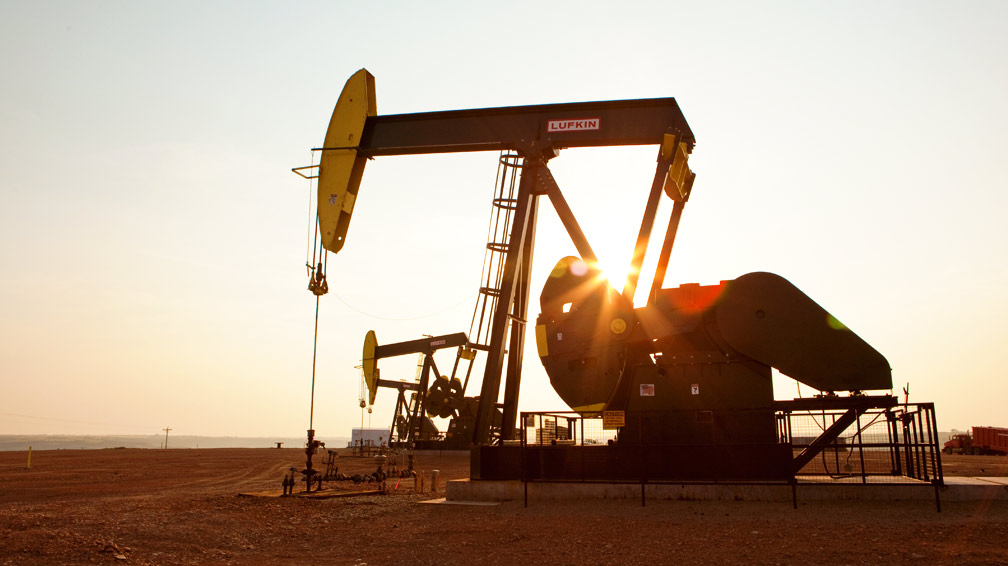The photograph captures a morning scene of an arid, reddish-brown desert landscape featuring multiple oil pump jacks. The central focus is a side view of an oil rig, characterized by its mechanical, crane-like design that operates with a seesaw motion. The rig features a horizontal black bar on top and a prominent yellow hammerhead structure on the left, which is connected to a rod that plunges into the ground. This rod is designed to extract oil, which is then presumably pumped through pipes at the base. To the left and in the background, there's another similar oil rig, and further back, the edge of a large red freight truck is visible on the far right. The ground beneath the rigs consists of flattened, reddish-brown dirt, and a solid concrete platform supports the main base of the front rig. Overhead, the sun is beginning to rise, casting beams of yellow light across the scene. The sky transitions from light yellow near the horizon to a pale bluish-green higher up, signaling the break of dawn in this vast, desolate environment.